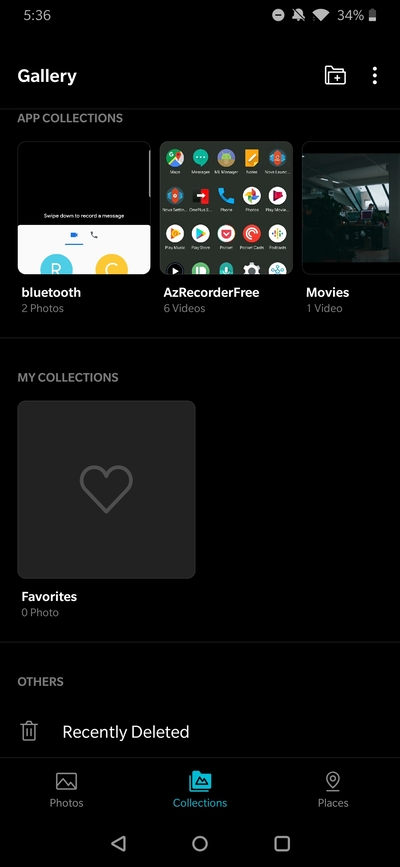This is a detailed screenshot from a phone's screen displaying the "Collections" tab within a gallery app. The image has a black background and shows the current time as 5:36 at the top left corner. On the top right corner, several status icons are visible, including a battery icon indicating 34% charge remaining.

At the upper left section of the screen, "Gallery" and "App Collections" are displayed. Under the "App Collections" heading, three categories are listed:
1. **Bluetooth** - 2 photos.
2. **AZ Recorder Free** - 6 videos.
3. **Movies** - 1 video.

Below these categories, there is a grayish-black square with a heart icon labeled "Favorites," which currently holds zero photos. In the "Others" section, a trash can icon signifies "Recently Deleted."

At the bottom of the screen, three navigation options are aligned side-by-side: "Photos," "Collections," and "Places." The "Collections" option is highlighted in blue, indicating it is the currently active tab. Finally, classic navigation symbols are centered at the very bottom of the screen: a white circle in the middle (home button), a white square to its right, and a back arrow to its left.

Overall, this is a detailed view of the collections interface within a phone's gallery app, showcasing various media categories and navigation options.